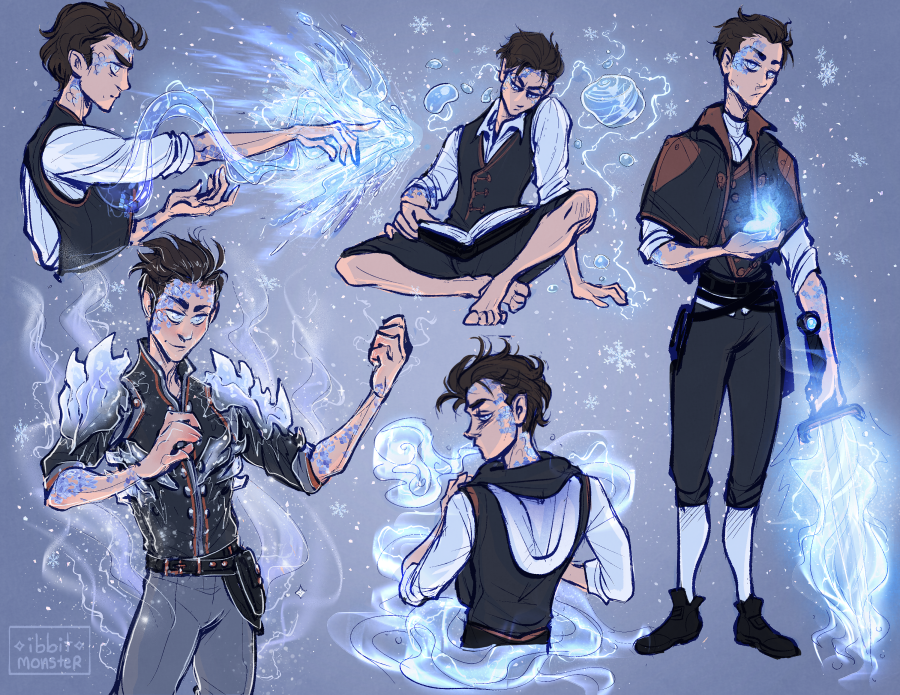The image depicts a detailed, multi-view drawing of a character, likely intended for a comic book or video game. The character appears Caucasian with distinct anime-style features, including large eyes that blend cartoon-like aesthetics with a hint of realism. He has short dark brown hair and a fair complexion. His attire consists of a black and brown jacket, gray shorts, long white socks, and black shoes. The character is illustrated in five different poses, each highlighting his supernatural abilities.

In the top left corner, he is shown pointing with bright white-blue flames streaming from his fingertips. To the right, the same pose is repeated, emphasizing his magical powers. The top center spotlights him sitting with his legs crossed, reading a book. On the far right, a full-bodied image shows him standing and holding a sword with blue flames emanating from it in his left hand, while his right hand holds another flaming object. The lower left view depicts flames coming off his shoulders, lending a dynamic sense of power. At the bottom center, the illustration focuses on his back, enveloped in smoke or flames, reinforcing his mystical inclination. The color palette includes blue, black, beige, brown, white, and shades of gray and lighter black, adding depth and texture to his overall look.